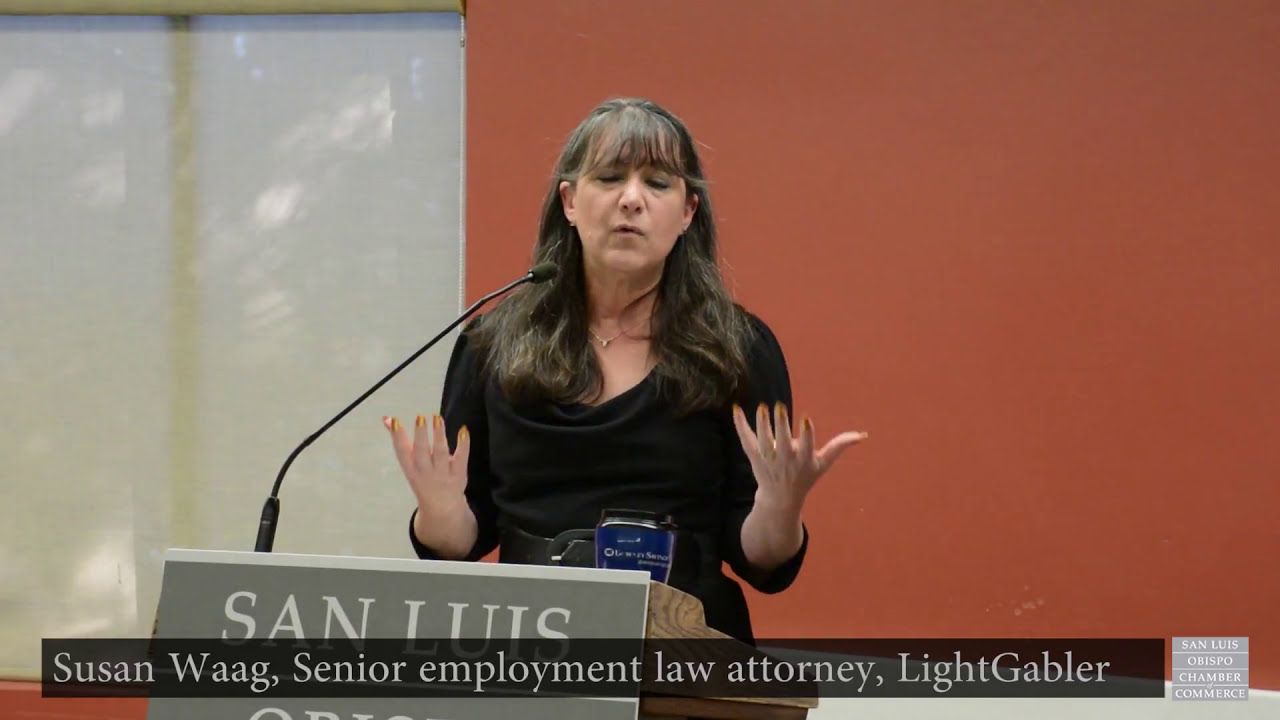The photograph depicts a woman with long, light brown hair and thin bangs, who is speaking at an event, likely a Chamber of Commerce meeting in San Luis Obispo. She is standing behind a wooden lectern, adorned with a gray name plaque. The plaque reads "San Luis" at the top, and below it, "Susan Wagg, Senior Employment Law Attorney, Light Gabler." The bottom right corner of the plaque mentions the "San Luis Obispo Chamber of Commerce." The woman, wearing a black long-sleeve shirt, holds her hands upward with her palms facing up, gesturing as she speaks. A thin microphone extends from the lectern close to her mouth, and a blue cup with a black lid and white writing rests on the right side of the lectern. Behind her, the background features a medium to salmon-colored wall, and to the left, there's a shiny whiteboard.